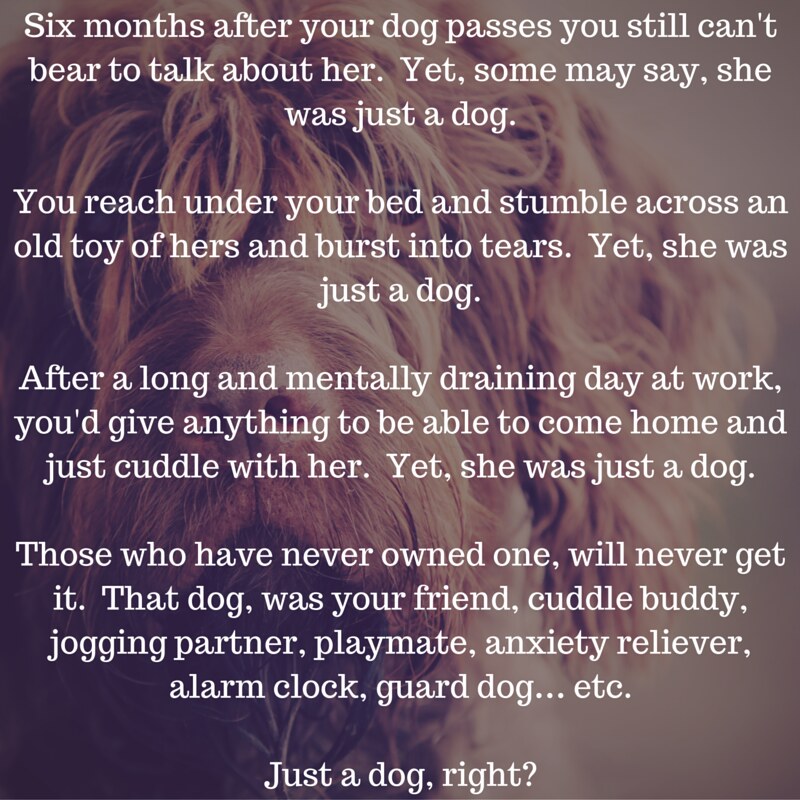The image features a poignant text overlay in white font, spread across four paragraphs, against a background picture of a poodle-like dog with light blonde or brown hair, partially visible through the text. The message reads: "Six months after your dog passes, you still can't bear to talk about her, yet some may say she was just a dog. You reach under your bed and stumble across an old toy of hers and burst into tears, yet she was just a dog. After a long and mentally draining day at work, you'd give anything to be able to come home and just cuddle with her, yet she was just a dog. Those who have never owned one will never get it. That dog was your friend, cuddle buddy, jogging partner, playmate, anxiety reliever, alarm clock, guard dog, etc. Just a dog, right?" The composition of text and image highlights the deep emotional bond between a dog and its owner, emphasizing that a pet is far more than "just a dog" to those who have loved one.